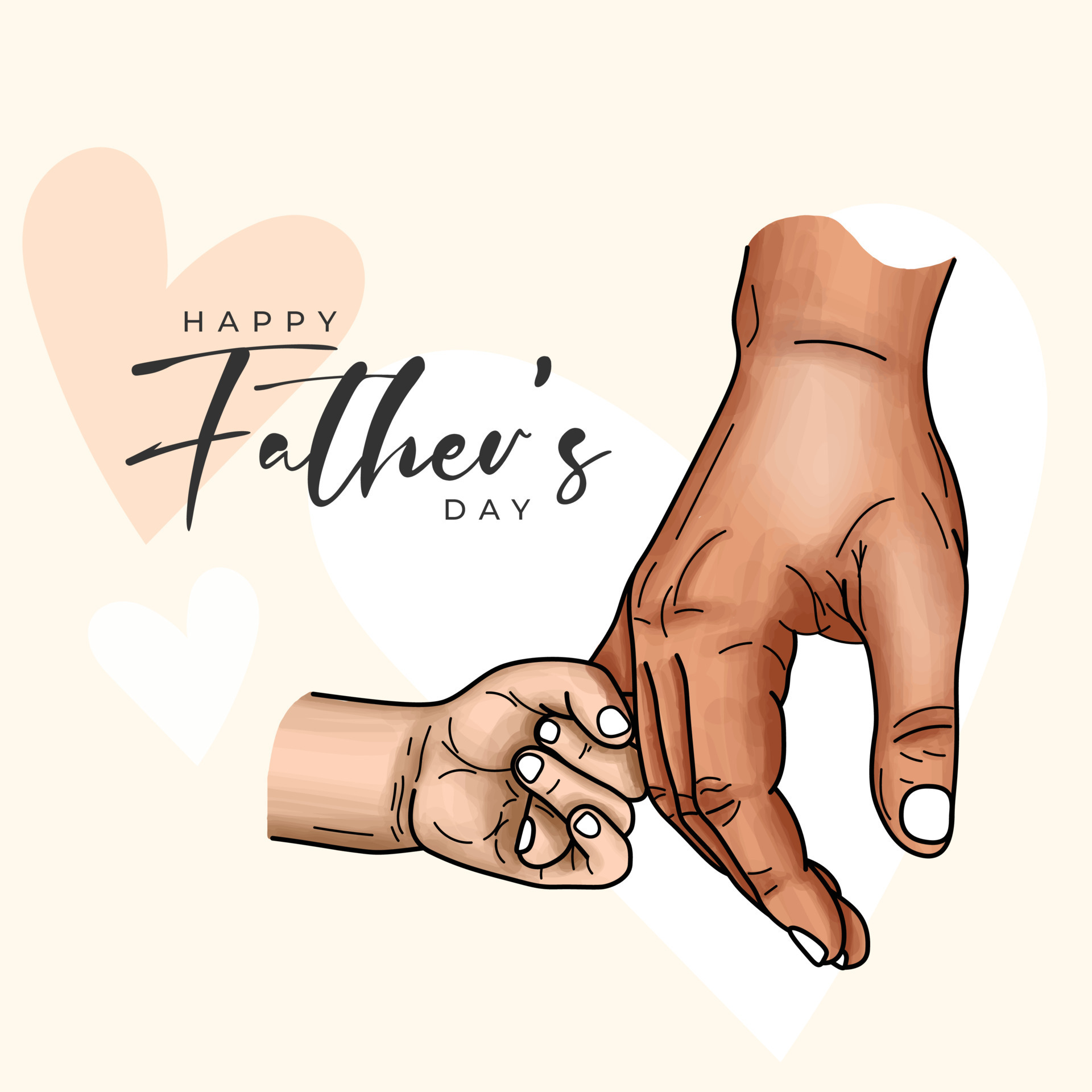This is a detailed graphic illustration, ideal for a social media post on platforms like Instagram or Facebook, celebrating Father's Day. It features a touching scene where a small child's light brown hand is clasping the pinky finger of a larger, darker brown adult hand. Both hands are prominently displayed against a large white heart situated on the right side of the image. Additionally, there are two other hearts to the left; one heart is a peach color while the other is white. The overall background of the graphic is a tan color, enhancing the warm and heartfelt tone. Overlaid on this poignant imagery is the message "Happy Father's Day" in black lettering, with the word "Fathers" in bold to emphasize the celebration. The detailed depiction of the hands, including the white nails and visible creases, adds a realistic touch that makes this graphic reminiscent of a heartfelt Father's Day card, possibly one from a daughter to her father.